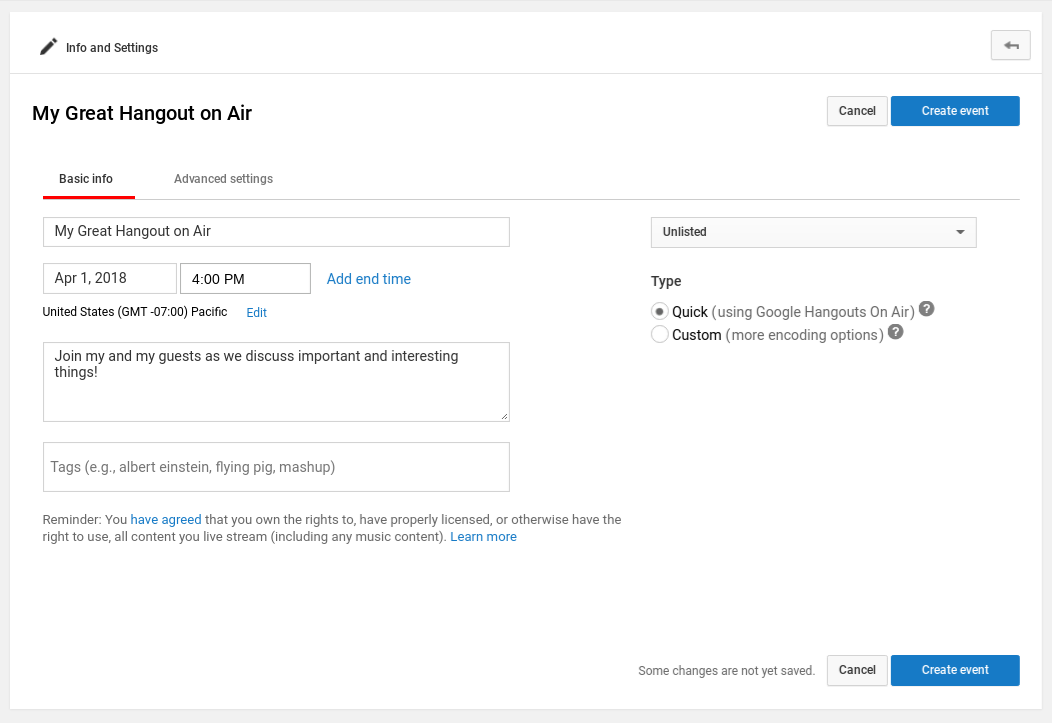The page features a clean white background bordered with a light gray margin at the top left corner. Positioned diagonally towards the bottom left is a gray pencil with the word "Info" printed on it, pointing towards an arrow that directs to left. On the far right of the page, enclosed within a light gray box with medium gray borders, there exists a divider marked by a bold black line. Above this divider, the text "My Great Hangout on Air" is prominently displayed in bold letters.

To the right of this text, there are two buttons. The first is a white "Cancel" button, and next to it, a blue rectangular "Create Event" button inscribed in white. Below these buttons are two tabs labeled "Basic Info" and "Advanced Settings." The "Basic Info" tab is currently selected, as indicated by a bold red line underneath it.

Users can interact with several editable fields on this page. The first field reads "My Great Hangout on Air." The next field states the date and time as "April 1st, 2018, 4:00 PM". To the right of this entry, a blue "Add End Time" link is available. Below this, small black letters spell out "United States (GMT-07:00) Pacific," accompanied by a blue "Edit" option.

Further down, another editable section prompts the user, "Join my guests and me as we discuss important and interesting things!" Exclamation mark included. Another field below this allows for text entry with placeholder text in gray reading "Tags (e.g., Albert Einstein, flying pig, mashup)." Beneath these fields lies a small note in very small gray font: "Reminder: You have agreed that you own the rights to, have properly licensed, or otherwise have the right to use all content you livestream, including any music content." The phrase "have agreed" is clickable and highlighted in blue, with a "Learn more" option available in blue as well.